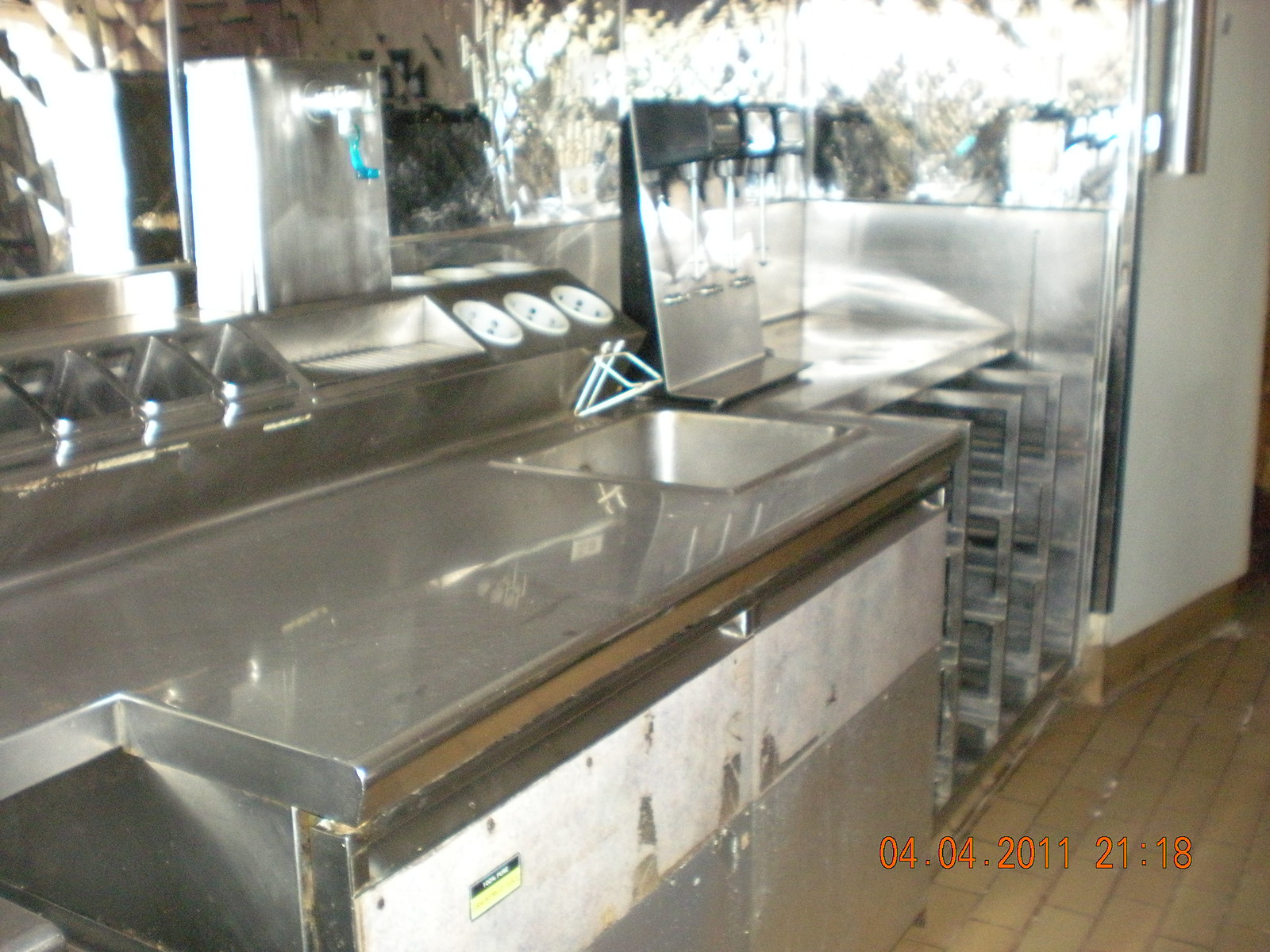The image captures a somewhat blurry snapshot of a commercial or industrial kitchen, likely from a restaurant or fast-food establishment. In the lower right corner, an orange timestamp reads "04 04 2011 21:18," indicating the date and time it was taken. The kitchen features stainless steel countertops and a single sink with a light blue faucet. Behind the countertop, there are three empty white caddies, potentially for silverware, along with visible stainless steel racks and small cubbies to the left. There is also a soda fountain dispensing machine in the background. The flooring consists of tan rectangular tiles laid out in a brick pattern, and a white kitchen door is located on the right side of the image. Despite its poor focus and somewhat blurry quality, the photo reveals a utilitarian and sparsely furnished space, brightly lit but devoid of any visible food items.